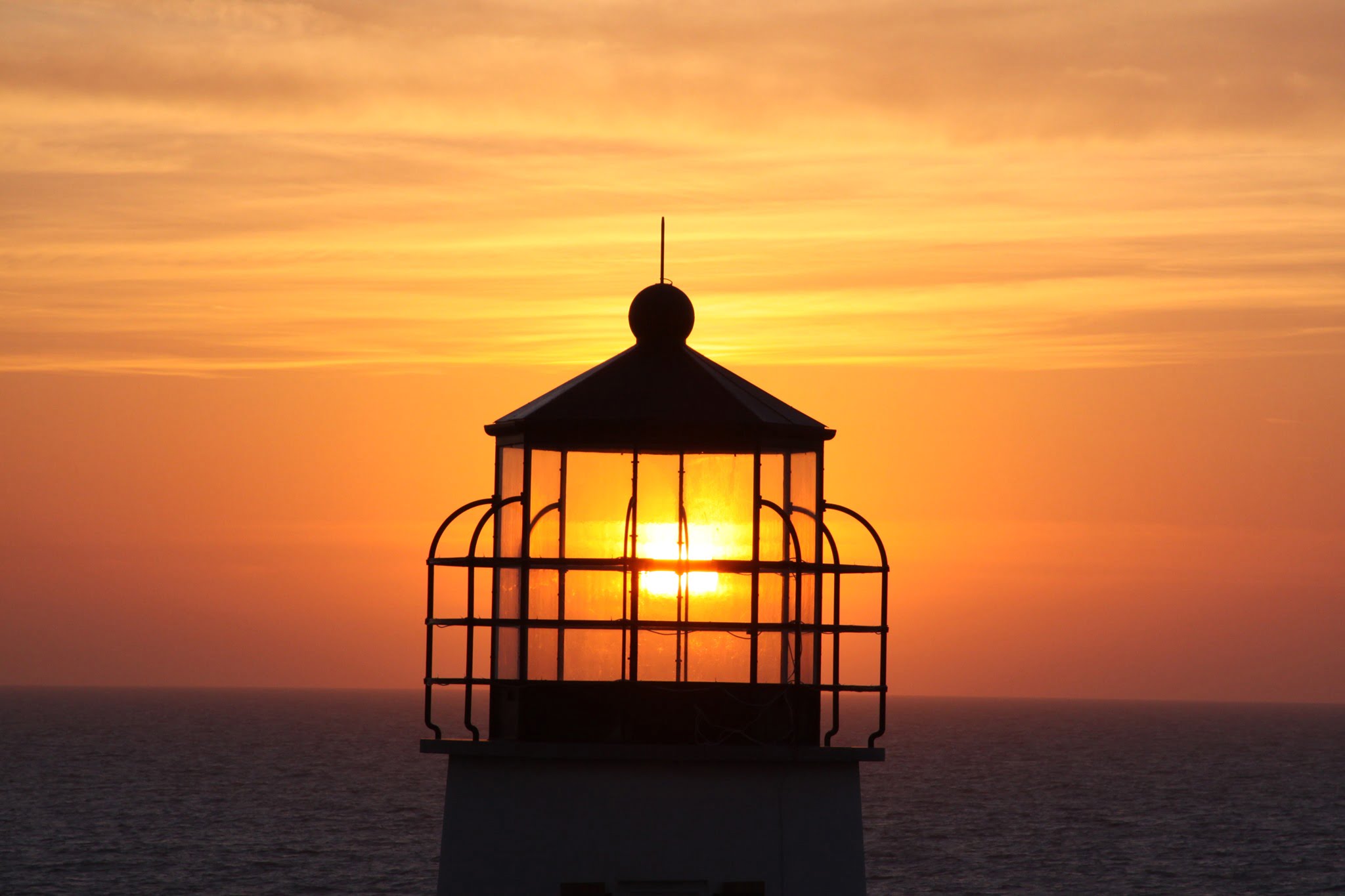The photograph captures the striking image of a lighthouse, primarily focusing on its top section, surrounded by protective guardrails. The lighthouse itself casts a shadow, enhanced by the glowing glass enclosure that hints at the light being turned on, with a warm yellow radiance. The setting appears to be during sunset, with the sky ablaze in hues of orange and yellow, with glowing clouds adding to the vibrant scene. Below the lighthouse, the ocean stretches out, depicted in a deep dark blue, almost merging with the blackness of twilight. The photograph is horizontally rectangular, devoid of a border, offering a clear, unframed view into this mesmerizing scene. The copper-looking roof and the cement structure of the lighthouse down to the ground add to its robust appearance. The light from the setting sun may be reflecting off the lighthouse's glass, creating a harmonious blend of natural and artificial light. The sunset showcases a dramatic gradient from purple at the horizon to lighter pink and ultimately gray, enhancing the serene and picturesque quality of the image. This outdoor photo vividly portrays the balance between the steadfast lighthouse and the ever-changing sky and sea, suggesting the work of a professional photographer aiming for a blend of artistic and travel photography value.